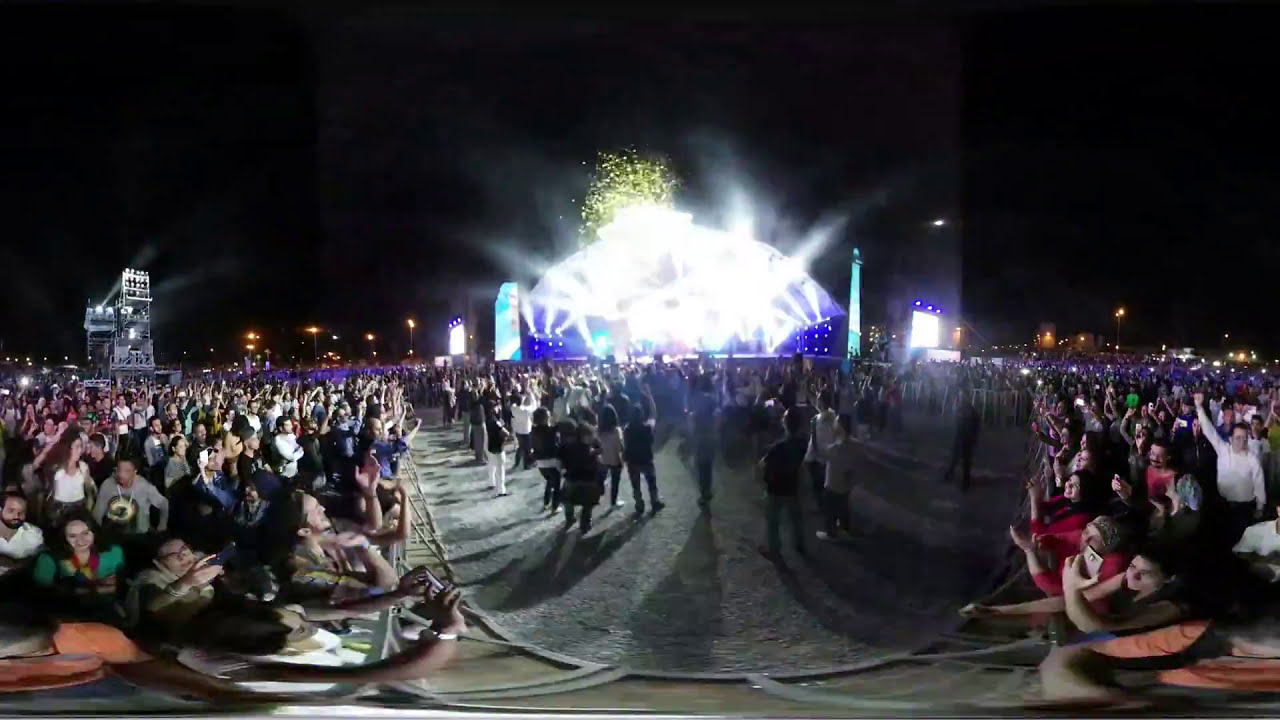This photo captures the electrifying atmosphere of a massive rock concert taking place at night. The scene is dominated by an extremely large and dense crowd of over 500 people, all tightly packed together, filling nearly every inch of space. The night sky above is pitch dark but is dramatically lit up by a spectacular light show emanating from the grand stage at the top of the photo. Bright, fantastic lighting pours out from the stage, featuring blue and white hues along with yellow fireworks that illuminate the scene. Additional towering lights shine towards the stage, creating a vibrant and dynamic visual effect.

In the center of the photo, the lighting creates the illusion of a semicircular area that's darker, possibly turning the crowd in that section into a striking black-and-white effect. This area almost gives the impression of people dancing on a carpet. To the left and right of this central zone, the sea of concertgoers is clear, with many facing towards the stage or the center of the image. Some individuals on the right have their hands raised, adding to the celebratory atmosphere.

The stage itself is lit up in stunning blue, with two prominent pillars glowing with blue and white lights. Fireworks are seen bursting at the back of the stage, enhancing the grandiose spectacle. The scene is further segmented by what appears to be barriers, dividing the crowd into three sections, adding an additional layer of structure to this vast, exhilarating music festival. The entire setup exudes excitement and energy as the crowd enjoys the live music and dazzling light show.